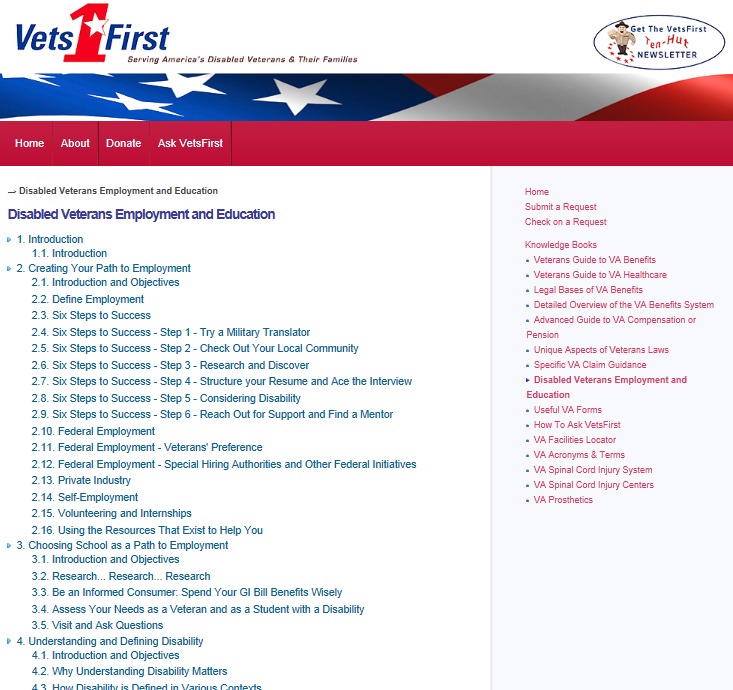The image showcases a web page dedicated to veteran services, prominently branded with "Vets First." A large red star and the text "Serving America’s Sailor Veterans and Their Families" draw immediate attention. Located on the right is an animated illustration of a man, set against a banner filled with stars reminiscent of the American flag. The website’s main menu includes options such as Home, About, Donate, Acts, and Vets First.

The header emphasizes "Disabled Veterans Employment and Education" in bold blue text. Below, there are several menu sections offering resources and guidance, including: 
1. **Introduction**
2. **Creating Your Path to Employment** (subdivided from 2.1 to 2.6)
3. **Choosing School as a Path to Employment** (subdivisions from 3.1 to 3.5)
4. **Understanding and Defining Disability** (subdivisions from 4.1 to 4.3, indicating further content to be added).

On the right side of the page, an additional menu provides options such as Home, Submit a Request, Check on a Request, and Books and Other Resources, offering further avenues for assistance and information for veterans and their families.